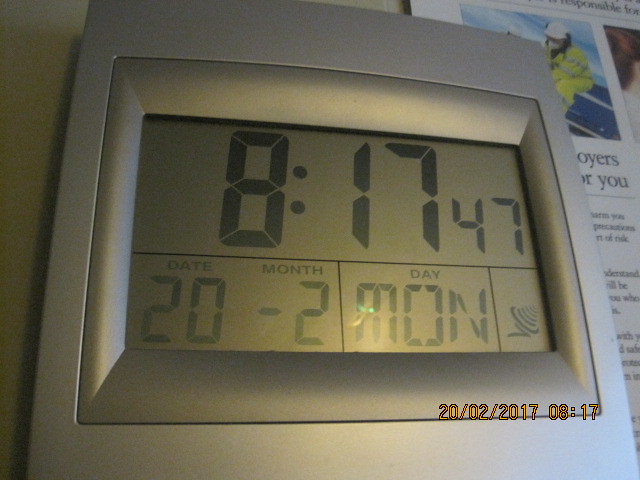This image features a silver digital clock prominently displaying the time as 8:17:47. The clock's digital display is square-shaped and encased in a sleek silver frame. The clock's face also shows important details; the date is set to the 20th of February, indicated as "20-2," accompanied by a possibly mistakenly added negative sign before the month. Below the date, the abbreviation "MON" denotes that it is Monday. Additionally, there is a graphic symbol indicating the volume level of the alarm. 

The clock appears to be either standing in front of or lying on top of a poster or article. The background shows an image of an individual wearing a yellow suit and a white hard hat. The photo capturing this scene was taken on February 20th, 2017, precisely at 8:17 AM.